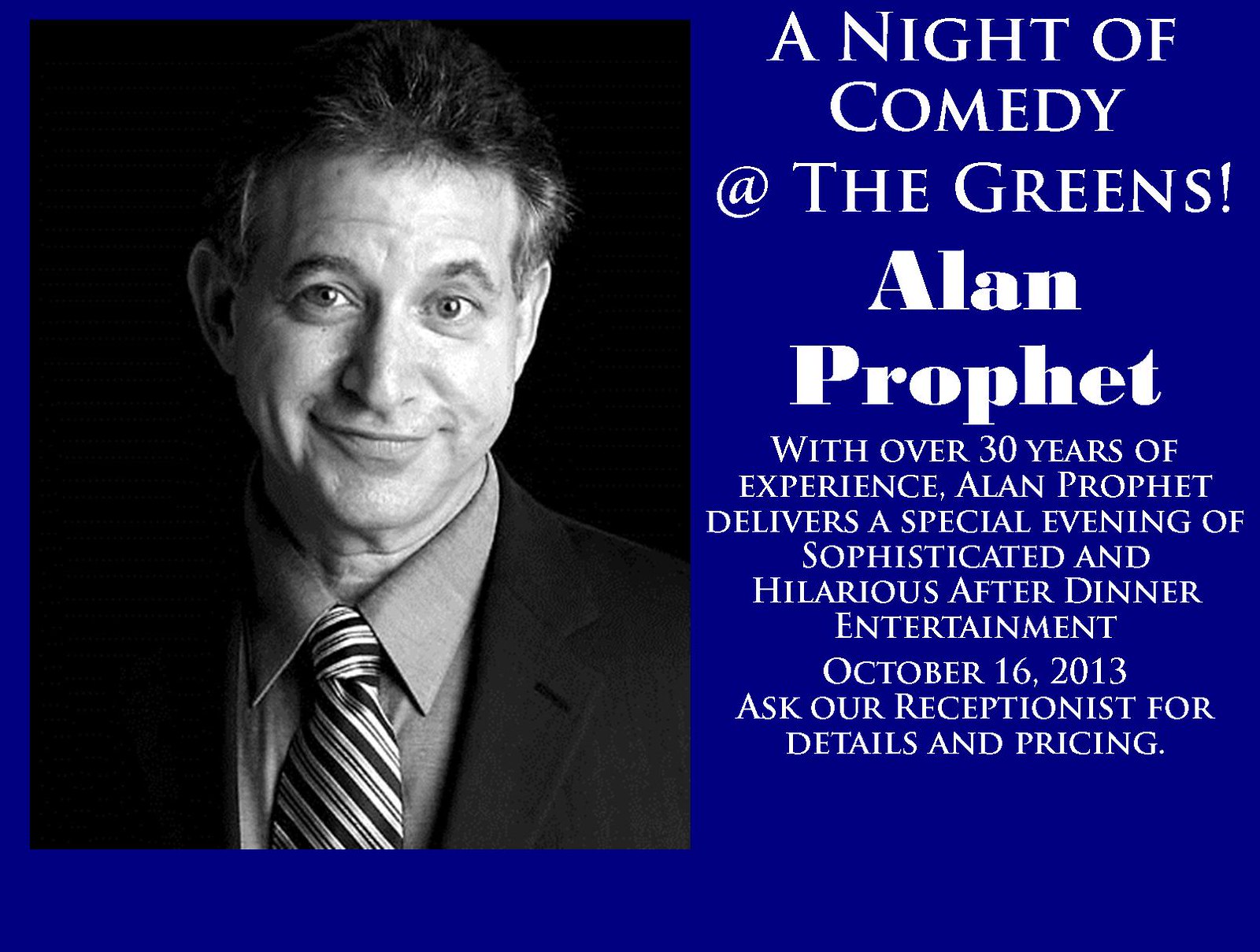This promotional flyer, set against a dark blue background, features a black-and-white headshot of a man with white skin and short, dark hair taking up the left half of the image. He is smiling and facing forward, dressed in a dark suit, a grey dress shirt, and a striped tie. The right side of the flyer contains white text detailing the event. At the top, it reads "A Night of Comedy at The Greens" in prominent white letters, followed by the name "Alan Proffitt" in bold. Below, it states, "With over 30 years of experience, Alan Proffitt delivers a special evening of sophisticated and hilarious after-dinner entertainment." The date of the event, "October 16, 2013," is then listed, with a note at the bottom advising, "Ask our receptionist for details and pricing."